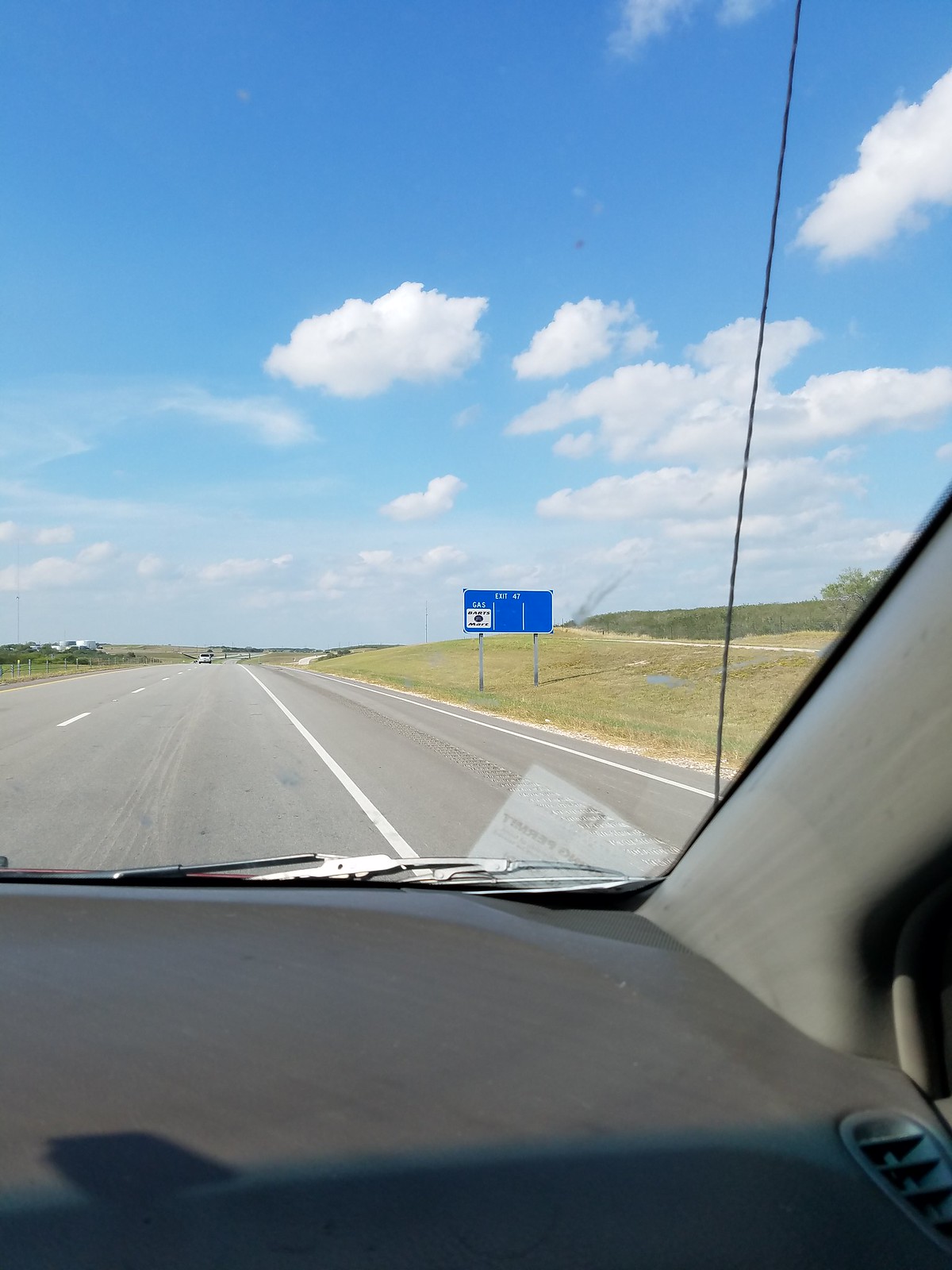A photograph taken from inside a moving vehicle on the passenger side shows a clear, unobstructed view of the highway. The bottom of the image captures part of the gray dashboard, slightly tucked down and shadowed, along with some paperwork resting at the front of the windshield. A windshield wiper and an aerial are visible, sticking out from the side. The concrete road ahead appears remarkably clear with only a single vehicle visible in the distance. The highway, marked with white dashed lines, spans three lanes that are largely empty. The roadside features patches of green grass, some of which look dried and dead. A prominent blue sign stands on the right side, though its text is unreadable. The sky above is a vibrant blue, transitioning from a darker hue at the top to a lighter one lower down, and dotted with numerous fluffy white clouds, particularly concentrated everywhere except for the upper left part of the sky.